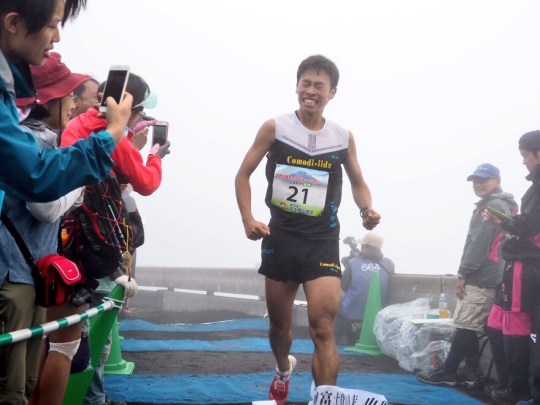The photograph captures the intense moment of an Asian runner crossing the finish line of a race, set against a slightly cloudy and foggy background that blends into a white, indistinct backdrop. The athletic man, clad in a black tank top with a white upper portion and black shorts adorned with yellow lettering, grimaces with his eyes closed and fists clenched by his sides, exuding pain and perseverance. His red tennis shoes stand out vividly against the three blue stripes marking the finish line on the road. The bib number "21" is prominently pinned to his chest. On his right side, a person in a pink jacket and a man wearing a blue hat can be seen, while on his left, a crowd of onlookers captures the moment with their phones, adding to the celebratory atmosphere. In the background, a photographer documents the scene, emphasizing the importance and magnitude of the event.